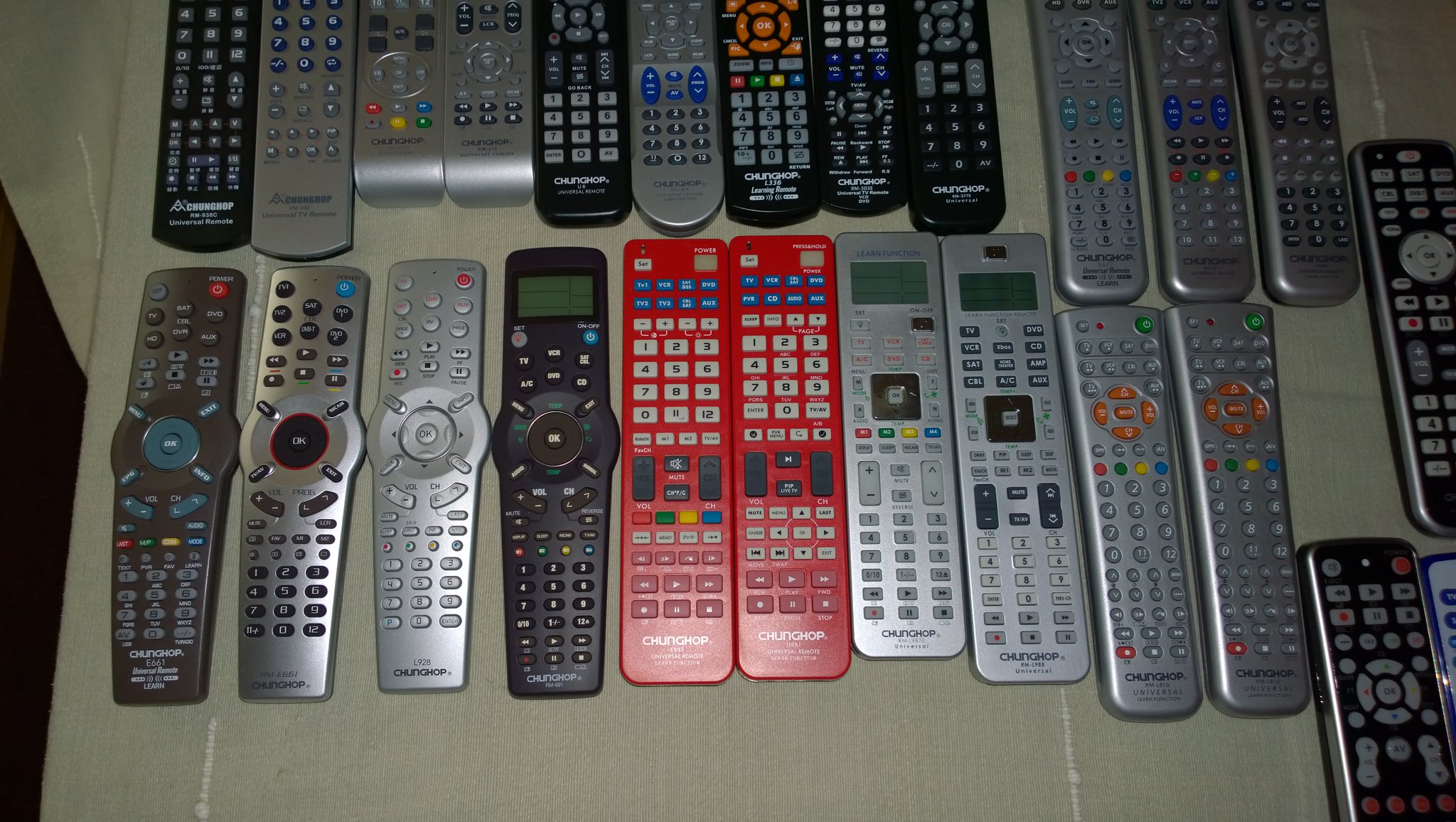The image depicts a wide-stretched landscape photograph showcasing an array of approximately 20 remote controls arranged on a surface that appears to be tiled, as suggested by the visible pale off-white grout lines. These remote controls, used for devices like satellite TVs, hi-fi systems, and traditional televisions, come in a variety of shapes, sizes, and colors. The collection features a mix of silver, dark grey, and a few distinctive red remotes, some with small LCD screens at the top.

The remotes are laid out in two primary horizontal rows, though the alignment isn't perfect. The bottom row consists of ten remote controls with an additional two slightly offset, summing up to twelve. The top row contains twelve remotes, with a thirteenth offset at the end. The remotes exhibit diverse designs: some are rectangular with rounded edges, some have a circular bump in the middle, and buttons of varying shapes and color schemes – from simple oblong buttons to squares and rounds, often color-coded for functionality. Among the notable features, two near-identical red remote controls stand out in the bottom row, distinguished only by the button colors.